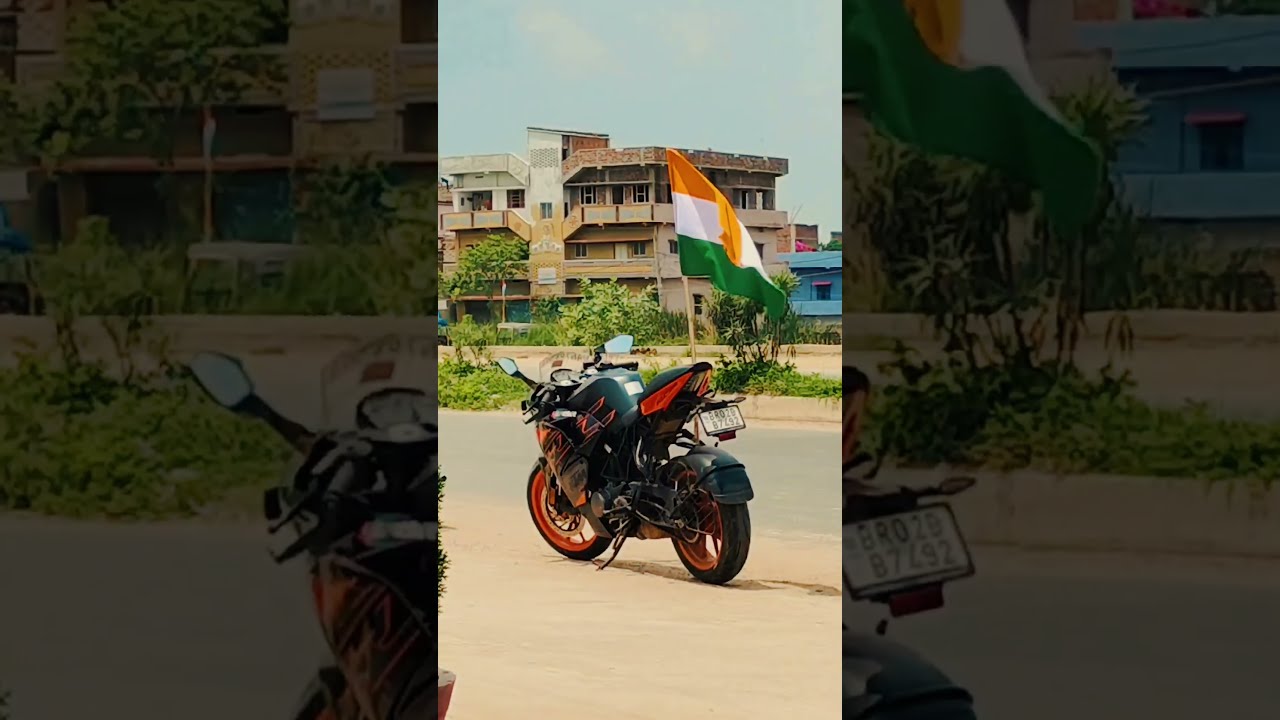In this detailed photograph, a stationary black motorcycle with red flame-like artwork and red-striped accents, including fenders and the inner rims of the wheels, is prominently featured in the foreground. A tricolor flag, potentially Mexican, with green, white, and red-orange horizontal stripes, is attached to the back of the motorcycle. The image is set on a sandy dirt road, indicating a seaside or beach-like location, with the kickstand clearly visible. Behind the motorcycle, low bushes and green grassy areas are present. Beyond these, there stands a multi-story building, likely seaside condos or apartments. The clear blue sky without a single cloud completes the serene background.